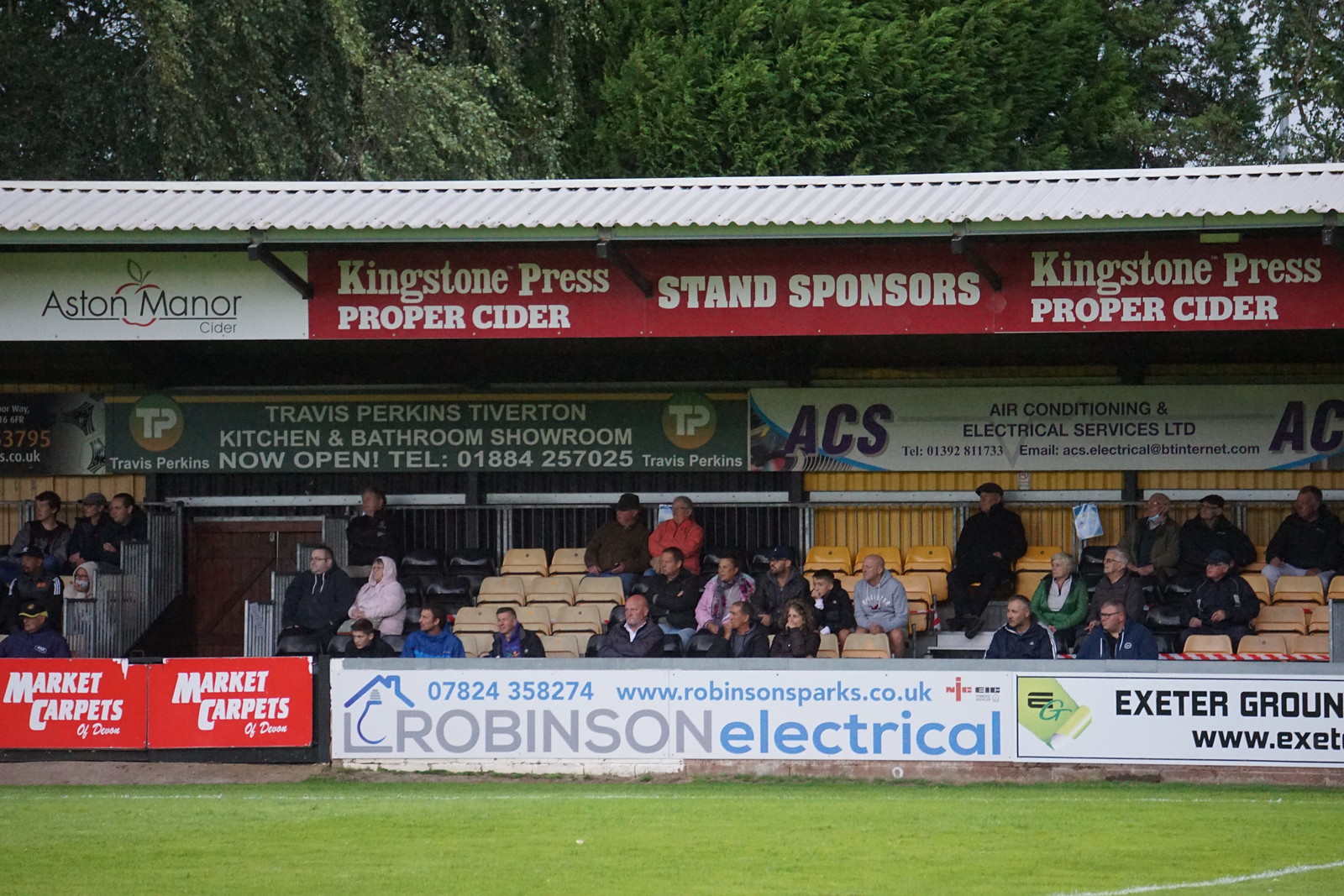This image captures a soccer stadium with half-filled bleachers, showcasing a mixed crowd of men, women, and children dressed in coats, indicating a chilly day. The stadium, surrounded by trees, features a visible soccer field and numerous advertisements. Prominently displayed sponsors include Robinson Electrical (with their website, www.robbinssparks.co.uk, and phone number 0782435827), Aston Manor Cider, Kingstone Press Proper Cider, and Market Carpets. Additional sponsors such as ACS (Air Conditioning and Electric Services Limited) and Exeter Ground also have signage visible throughout the venue.